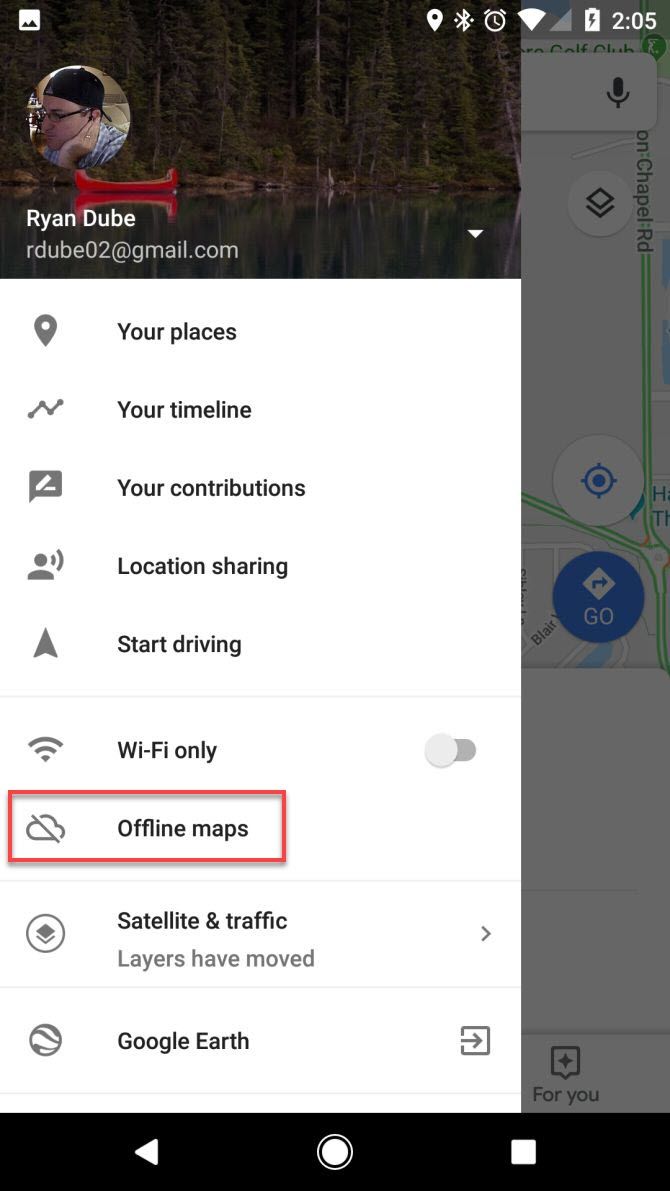A screen capture from a mobile device displays a user profile interface. Dominating the left side of the image is a profile picture of a person wearing a black baseball cap turned backwards. Behind this person's head, one can discern a scenic background featuring trees, a lake, and a red boat. Just below the profile image is the user's information: the name Ryan Dube is listed alongside the username rdube02 and the email address rdube02@gmail.com.

The interface also presents several selectable options arranged vertically beneath the profile information. These options, from top to bottom, include: 'Your Places,' 'Your Timeline,' 'Your Contributions,' 'Location Sharing,' 'Start Driving,' and 'WiFi Only.'

On the right side of the image, partially obscured by the profile and options, there is a map, hinting at the application’s navigational functionalities. The layout clearly separates the profile management features on the left from the map and navigational elements on the right.